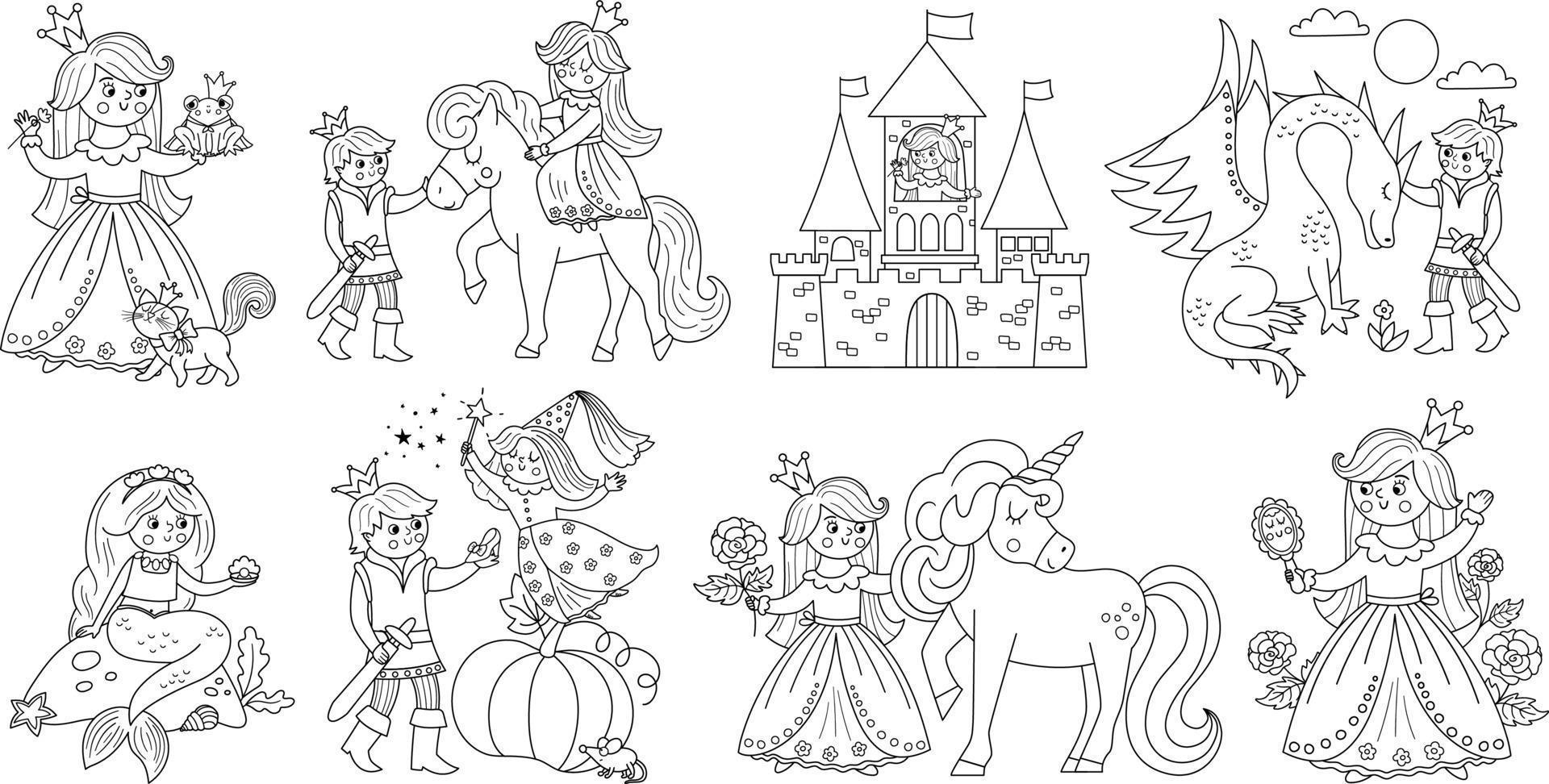This image features a page from a children's coloring book, designed with several intricate and uncolored line drawings, intended for children to color in. The page is divided into two rows with four images each, making a total of eight distinct illustrations. 

On the top row, the first image depicts a princess holding a frog, with a cat by her side. The second image shows a princess riding a horse while a prince gently pets the horse's nose. The third image portrays a princess gazing out from within a castle window. The fourth image highlights a prince petting the head of a friendly dragon.

On the bottom row, the first image features a mermaid holding a seashell while sitting on a rock. The second illustration is a fairy tale scene with a prince holding a glass slipper while the princess, standing on a pumpkin, waves a magic wand, a nod to the story of Cinderella. The third image shows a princess lovingly petting the mane of a unicorn and holding a flower. The final image illustrates a princess looking into a mirror, surrounded by flowers, reflecting a happy expression.

These detailed black-and-white line drawings encompass enchanting themes of princes, princesses, mythical creatures, and magical scenes, typical of a children's fantasy coloring book.